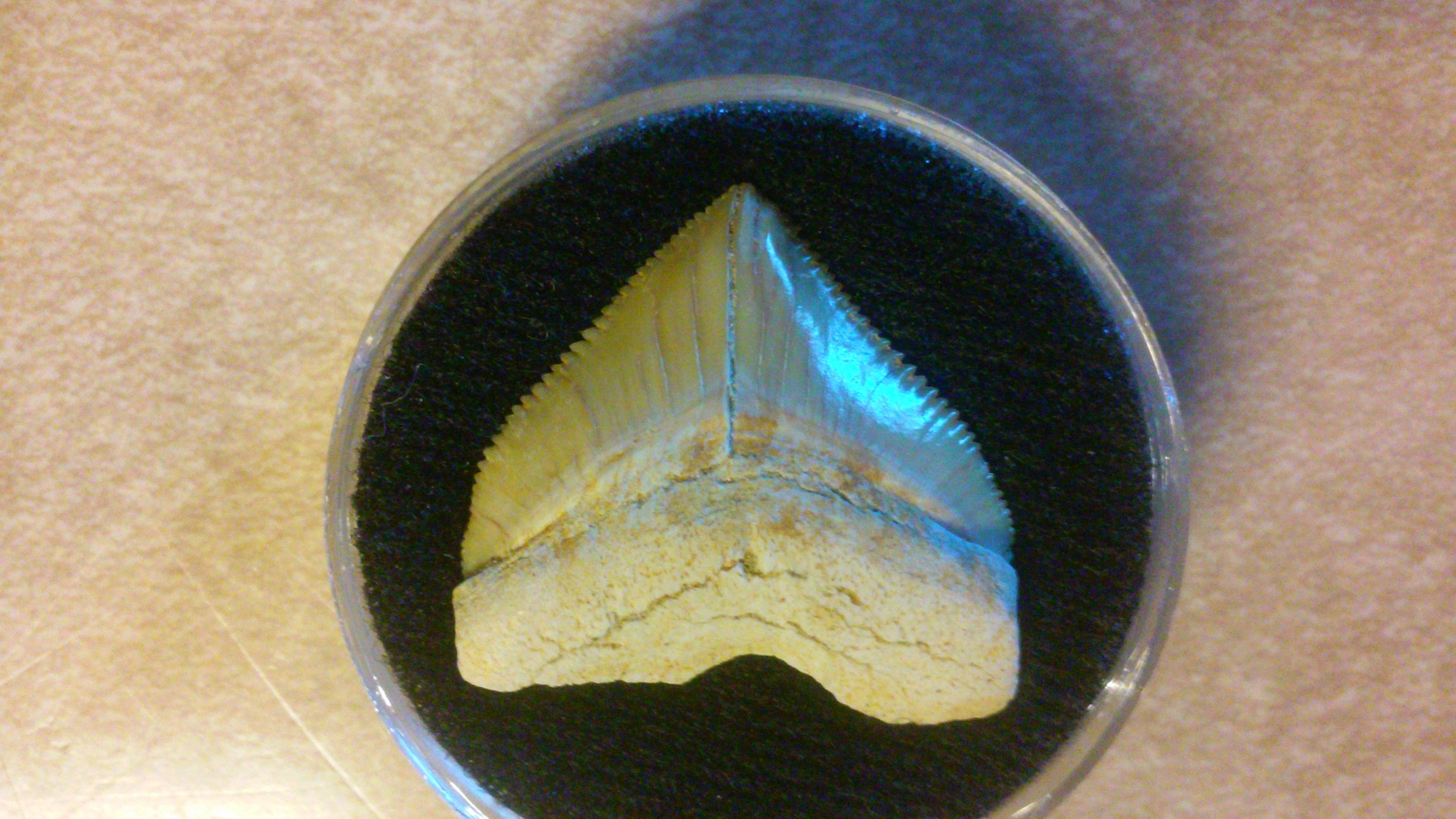The image depicts an abstract composition centered on a craggy and cracked stone fin resting in a glass bowl, set against a reddish-white background. The bowl contains a black object that could be interpreted as padding, elevating the stone fin which is smooth at the top with many sharp points converging to a central peak. Surrounding details offer various interpretations, suggesting the fin could resemble a bone or fossil due to its irregular, ivory-hued surface with touches of pale brown and gold. The background might be a peachy, fleshy-colored surface, creating a stark contrast that frames the glass dish containing this mysterious artifact. The fin’s unique texture and color make it a focal point that could evoke imagery of a shark tooth or a beak, positioned within what might initially appear to be artificial turf or cushioning inside the bowl.